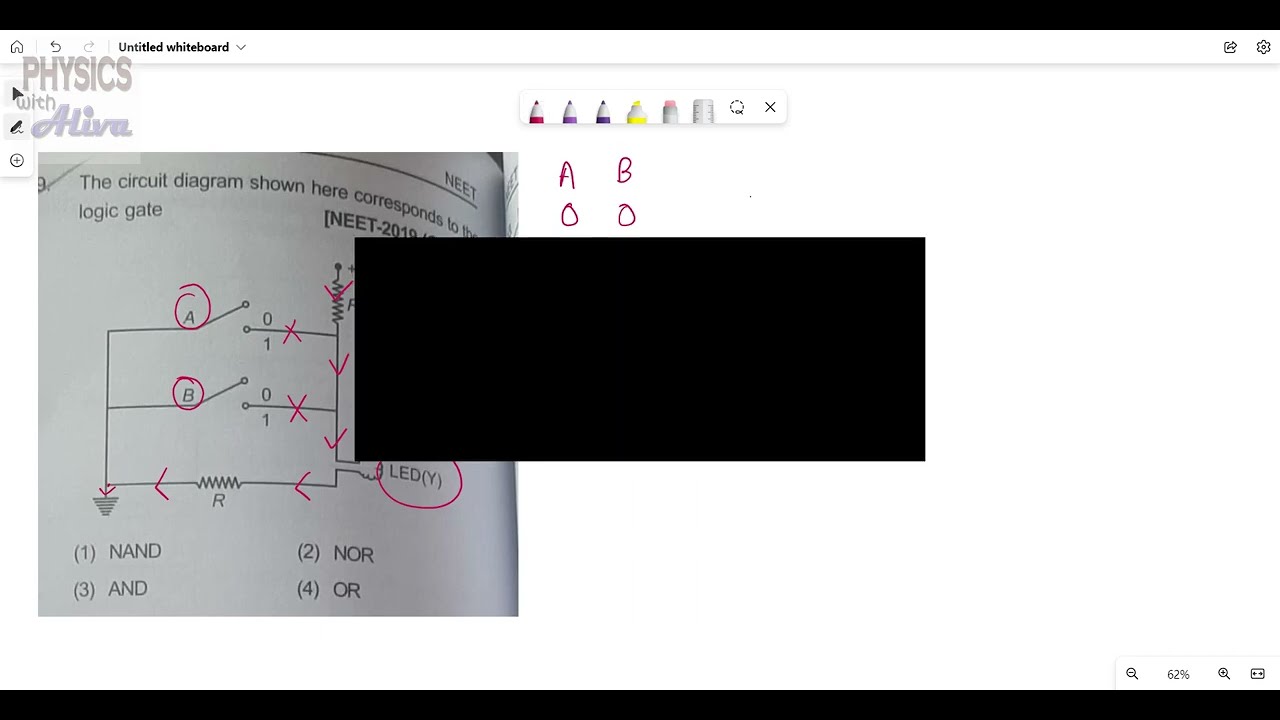This image appears to be a screenshot of a digital whiteboard labeled “Physics with Aliva” in the top-left corner. The whiteboard displays a page from a book featuring a detailed circuit diagram relevant to logic gates. In the center of the screen is a prominent black rectangle, partially obscuring the underlying content. Below this, the diagram lists the terms "1. NAND, 2. NOR, 3. AND, 4. OR" as potential types of logic gates. The circuit drawing on the left side of the screen includes a representation of a bulb, wires, and symbols like a circled 'B,' 'X,' 'LED,' and 'Y,' while labels 'A' and 'B0' stretch vertically near the center black box. Additional markings such as a resistance symbol, connectors, and NEET-21 can be seen towards the top-right corner. Various tool icons, including markers, an eraser, an undo symbol, and an 'X,' are aligned at the top, suggesting a digital workspace for solving complex physics problems involving logic gates.